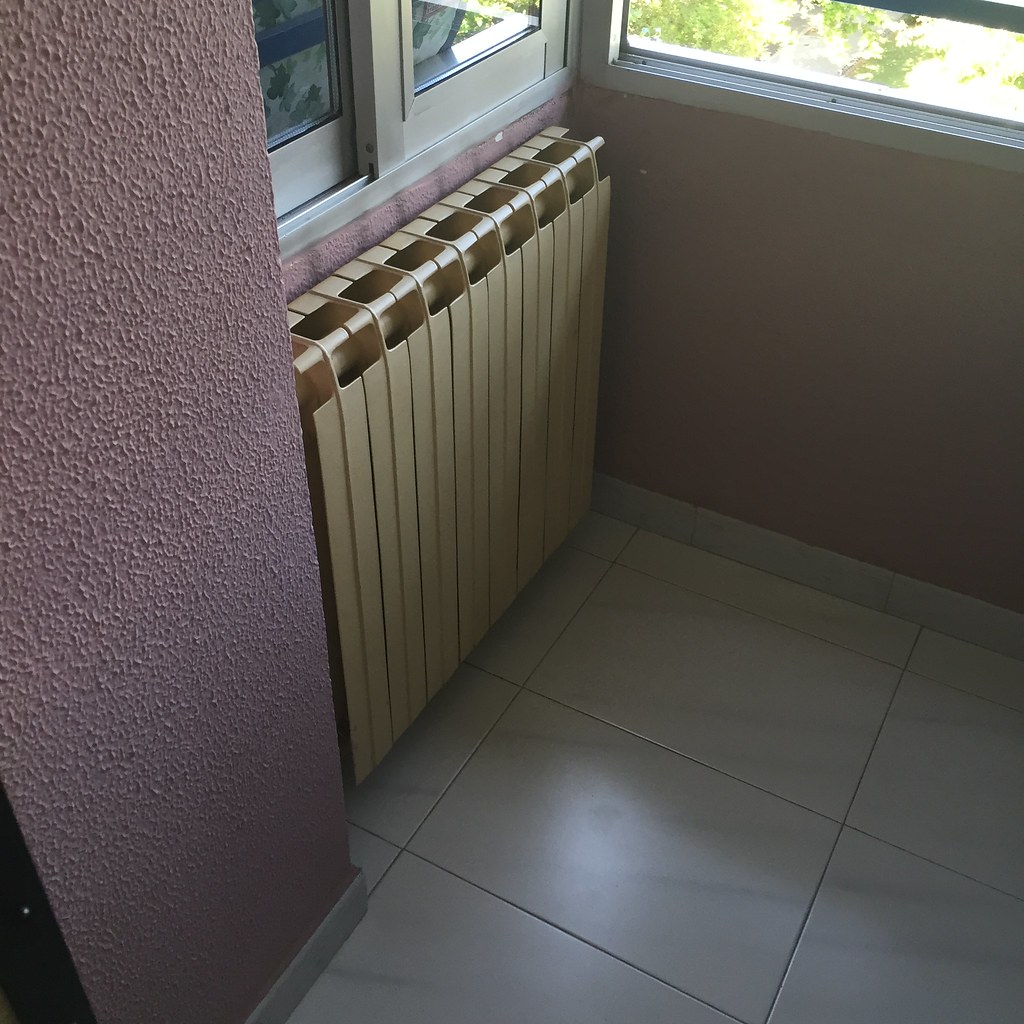This photograph captures a corner of an indoor space, featuring distinctive pink stucco walls bathed in sunlight. The upper right corner showcases a window revealing a clear, sunny day with lush green trees outside. On the left side, another window partially visible near the bottom has a bamboo-like air conditioning unit attached beneath it. The floor is covered in white marble tiles streaked with gray, adding a touch of elegance. Both windows are framed in stainless steel, giving a modern flair, with the window on the right lacking any screen. Centrally located below the windows is an old-fashioned, beige-colored radiator or air conditioning vent, tucked into a small alcove. The overall setting feels more like an office or a business space, complemented by its polished tiles and meticulous metal trims around the windows and floors.